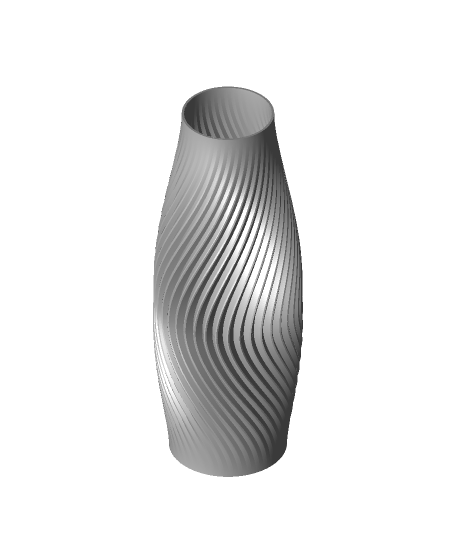This image depicts a tall, slender, modern gray vase with a distinctive wavy design etched across its surface. The waves start at the top, curve leftward, and then undulate rightward, giving it a dynamic appearance. The vase exhibits a grayish-silver hue and has a smooth, even opening at the top while expanding slightly towards the base, ensuring stability for standing upright. The overall silhouette resembles a blend of a bulging bowling pin and a coke bottle, with a gracefully curving middle. Set against a completely white background, the texture of the vase suggests it could be ceramic or digitally rendered, highlighting its ornamental and artistic appeal. Perfect for holding flowers, the vase blends functionality with aesthetic charm, featuring no text to distract from its modern, minimalist style.